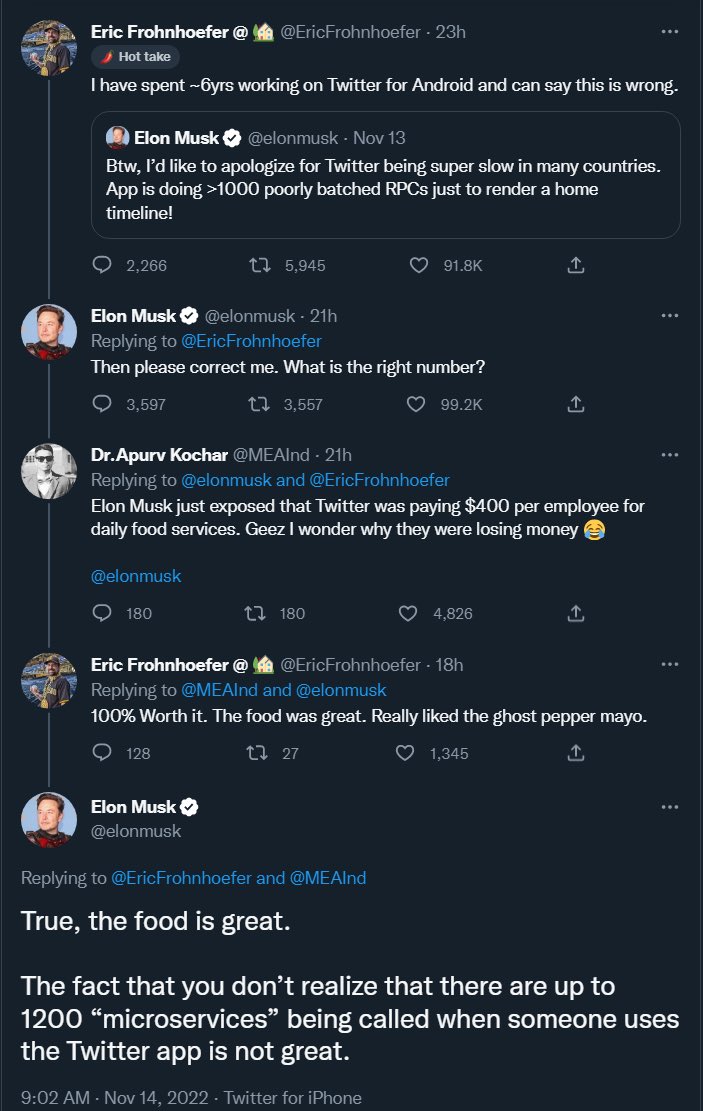In the screenshot, we observe a section of social media posts against a solid black background, with white text prominently displayed. The focal point is a post by Eric Fraunhofer, evidenced by the included image of him, a man who appears to be in his 40s, wearing a cap, with a beard and mustache, and fair skin. Eric's post is labeled "hot take," accompanied by a chili pepper emoji, indicating a strong opinion. He claims with authority, "I have spent six years working on Twitter for Android and can say this is wrong."

Above Eric's post is a tweet from Elon Musk, dated November 13th, where he apologizes for Twitter's slow performance in many countries, attributing the issue to the app making over 1,000 poorly batched RPC (Remote Procedure Call) requests just to render a home timeline. This tweet has garnered significant interaction, with 2,266 replies and 91,800 likes. 

Below Eric's post, there is a subsequent reply from Elon Musk, directly addressing Eric's critique, in which Musk, verified by a blue checkmark, questions, "Then please correct me, what is the right number?"